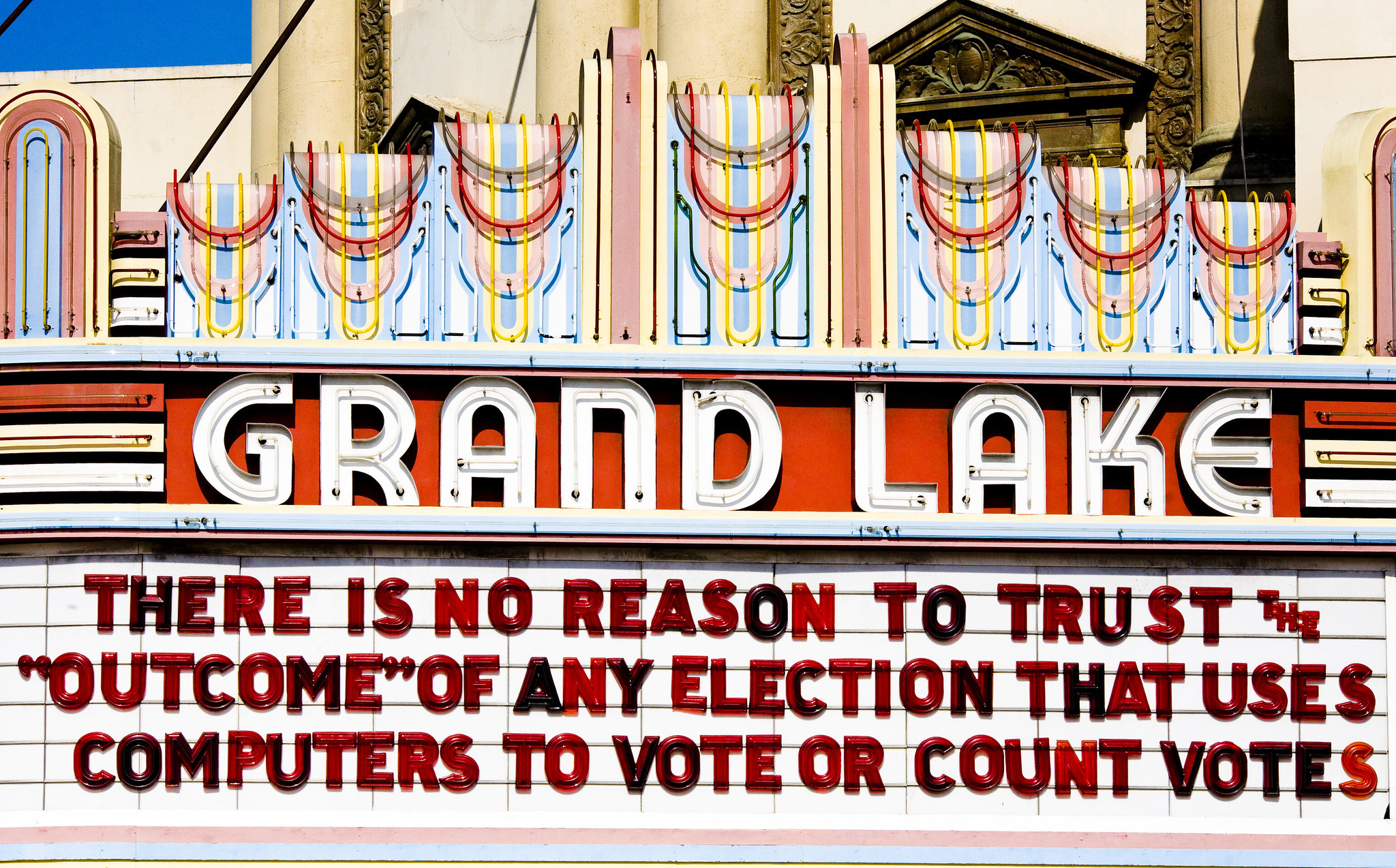In this full-color photograph, we see an old-fashioned movie theater marquee sign, set against a daytime sky. The sign prominently displays the name "Grand Lake" in bold white letters against a vibrant red panel with a blue trim. Above the name, several decorative, looping neon lights—likely capable of flashing in various colors at night—enhance the vintage charm of the marquee. Beneath "Grand Lake," a red sign with removable tiles and black letters states, "There is no reason to trust the outcome of any election that uses computers to vote or count votes." The scene includes a light beige concrete building with round pillars, adding to the nostalgic atmosphere of the outdoor setting.